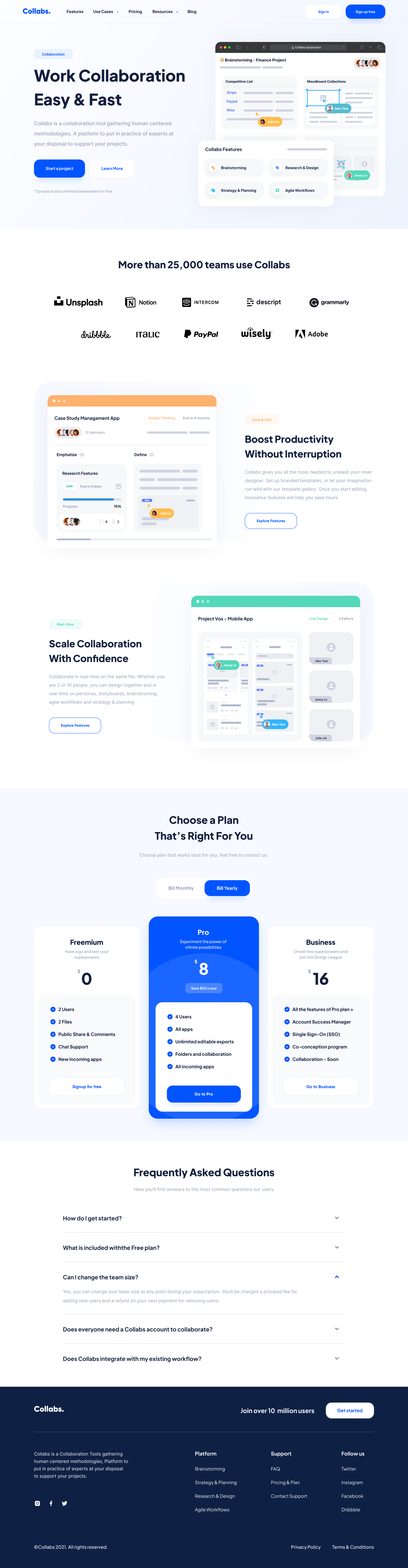A narrow and elongated image features a website layout designed for collaboration tools. 

### Top Section
- **Header**: On the top left is the word "Collabs" in dark blue text on a white background. To the right are five text headings: "Features," "Use Cases" with a dropdown arrow, "Pricing," "Resources" with a dropdown arrow, and "Blog."
- **Main Action Area**: 
  - The section beneath the header reads "Collaborations" in blue, and underneath that, "Work Collaboration Easy and Fast" in black. 
  - There's a paragraph of smaller black text explaining more about the tool.
  - Two primary buttons: a blue "Start a Project" button and a white "Learn More" button beside it.

### Upper Right Section
- **User Options**: 
  - A white button with "Sign In" in blue letters and a blue button with "Sign Up Free" in white letters.

### Mid Section
- **Small Interactive Window**: 
  - A window with a dark grey border at the top, featuring red, yellow, and green dots on the left. The center text is small and unreadable, in white lettering, along with white icons at the top right.
- **Project Information**: 
  - "Brain Brainstorming Finance Project" in black text, accompanied by user icons on the right side of the white background.

### Competitive Features List
- **Platforms**: 
  - A section listing "Stripe," "PayPal," and "Wise," with an orange button at the bottom.

### Mood Board
- **Mood Board Collection**:
  - A turquoise button with white lettering.

### CoLab Teachers
- **Instructional Area**:
  - A white window with "CoLab Teachers" written in black. 
  - Four grey buttons: 
    - Top left: "Brainstorming"
    - Top right: "Research and Design"
    - Bottom left: "Strategy and Planning"
    - Bottom right: "Agile Workflow"
  - In the far bottom right corner, a green button with white text, possibly reading "Jenny Lowe" or "Jeffrey Lowe."

### Lower Section
- **Testimonials & Usage Stats**:
  - Various windows promoting "Scale Collaboration with Confidence" and "Boost Productivity without Interruption."
  - Over 25,000 teams use CoLab, including icons of companies such as Unsplash, Nation, Intercom, Descript, Grammarly, Adobe, Wisely, PayPal, Italic, and Dribble.

### Pricing Information
- **Pricing Plans**:
  - Three vertical rectangles detailing what’s included in the free, pro, and business versions, along with their respective prices.

### Bottom Section
- **Footer**:
  - A large black panel listing multiple resources including FAQ, Pricing and Plans, Strategy, Sitemap, and Social Media Icons.

This well-structured image effectively communicates its purpose and offerings with clear headings, call-to-action buttons, and detailed sections for different features and pricing plans.